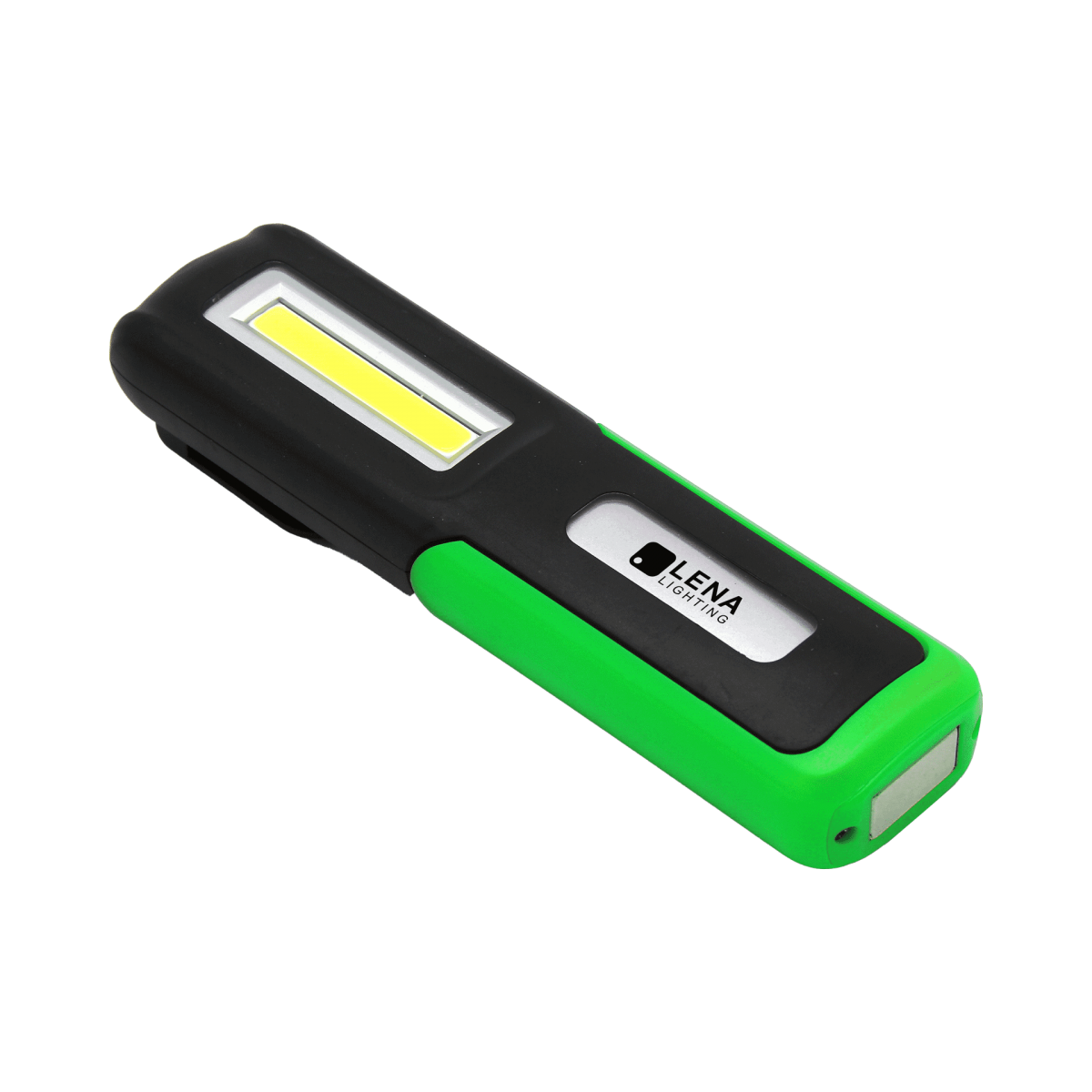The image is a sharp, color photograph of a long, thin, rectangular electronic device, oriented diagonally from the upper left to the bottom right, over a white or transparent background. The device, which appears to be a wireless workshop light from Lina Lighting, features a lime green bottom section and a black upper section with a gradient transition. It has a distinct, glowing yellow rectangular digital display or window at the top, bordered by a chrome lining. The bottom of the device includes a white rocker switch and a small hole, and features a silver rectangle labeled "Lina Lighting" with a black logo and square adjacent to it. The object, captured with photographic realism, is depicted as floating against the white background.